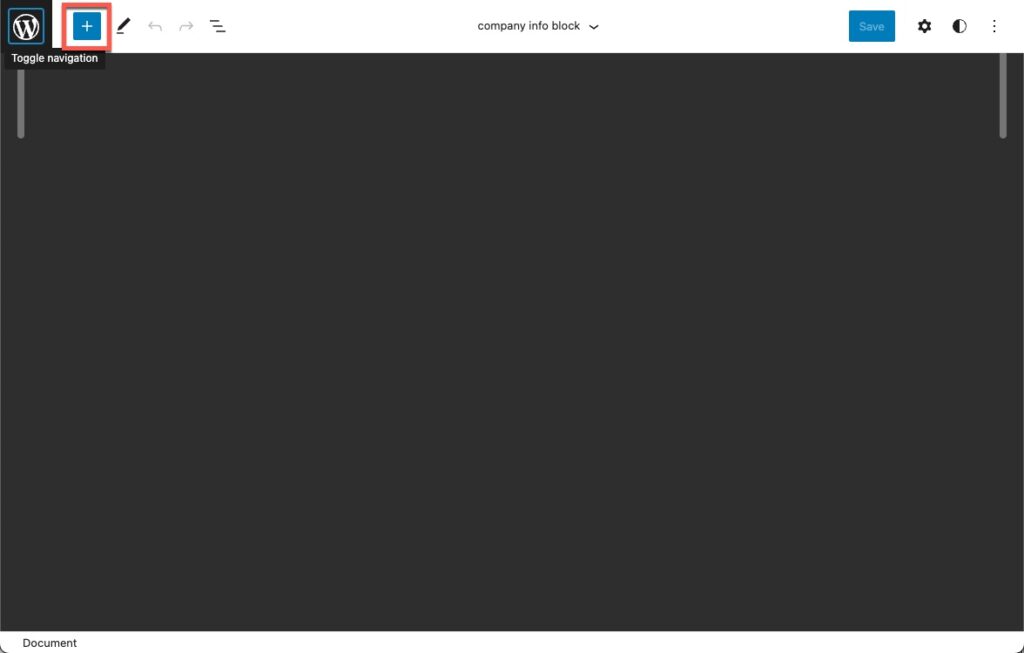An image depicting a user interface on a blank screen, with a detailed header section containing various icons and elements. 

At the top left, there's a black square featuring an inner teal square with a white-outlined circle inside, which encloses a white letter "W". Adjacent to this is a blue box with a white outer rim and a red trim, containing a plus sign. To the right of this box, there’s an icon resembling a crayon, and two arrows pointing left and right, respectively. Below these icons, angled downward from left to right, are three lines labeled "Company Info Block", which include a dropdown menu.

On the far-right end of the header, there's a blue save button, a gear icon indicating settings, and a circle divided into a black and white semicircle. Additionally, there are three vertical dots in the extreme right corner. 

Under the row of icons on the left, it reads "Toggle Navigation" in very small text, followed by a gray vertical line.